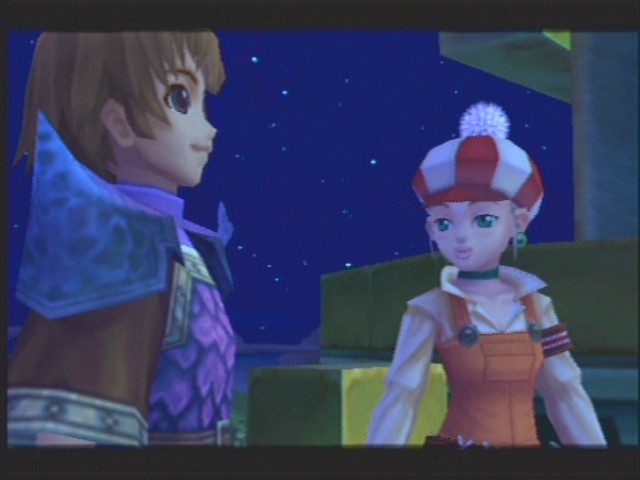This is a detailed screenshot from an anime-style video game set against a dark, star-strewn night sky. On the right side of the image stands a young girl with green-blue anime-like eyes and a heart-shaped face adorned with full pink lips, smiling gently. She wears a distinctive red and white hat with a white pom pom on top and two blonde strands of hair peeking out from under it. Her outfit includes green circular earrings, a green choker, a white long-sleeved shirt, and orange overalls. Behind her, colorful blocks are stacked, including a yellow square block with a green rectangle atop it. On the left side, a young boy with shaggy brown hair and large brown eyes is shown in profile, also smiling. He wears an armored-like attire featuring blue shoulder pads, a purple and blue chest plate, brown sleeves with silver edging, and a blue cape with a white border around the arm. The scene is evocative of early 2000s anime video game aesthetics.